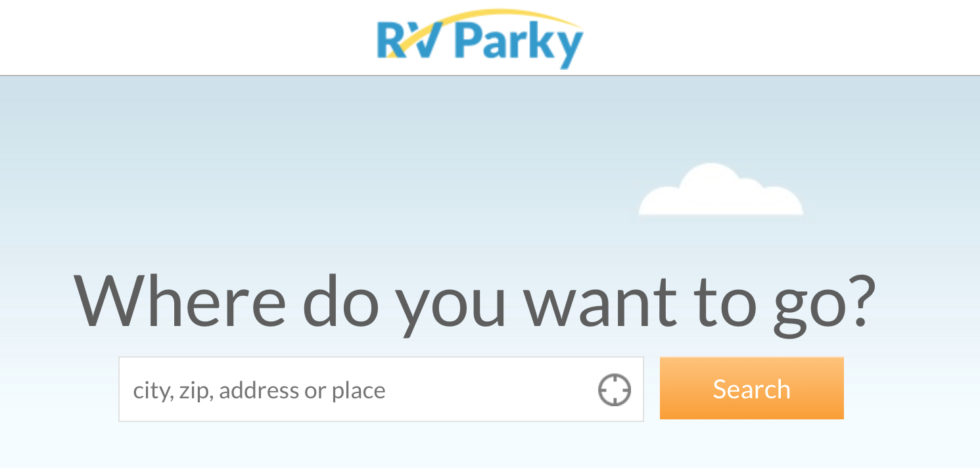The image showcases an attractive RV parking advertisement, predominantly featuring a visually engaging design with vibrant colors. 

At the top, the text "RV Parking" is prominently displayed in blue. A dynamic yellow swooping arc starts beneath the 'R,' gracefully extending through the 'V' before continuing its curve over the word "Parking" and ending near the 'Y.' This arc adds a sense of motion and draws the viewer's attention across the entire heading.

Below this, there is a sky-blue rectangular box, reminiscent of a cartoon-style clipboard. Inside this box, a single white, fluffy cloud is visible, enhancing the playful aesthetic of the image. Beneath the cloud, in bold black text, a large question reads: "Where do you want to go?" This inquiry is centrally located and encourages viewers to engage directly with the content.

Below the question, instructions are provided in smaller text, indicating that users can search for a city, ZIP code, address, or place, ensuring clarity on how to utilize the search function. Positioned to the right, a circular navigation icon provides additional emphasis on the search capabilities.

A prominent orange search button, with the word "Search" in white text, stands out at the bottom, designed to catch the eye and prompt immediate action from the user. This button's vibrant color contrasts effectively against the blue box, ensuring it is easily noticeable.

Overall, the white background of the advertisement maintains a clean and organized look, while the colorful elements strategically guide the viewer's eyes from the intriguing swooping arc, through the inviting question, down to the actionable search feature.